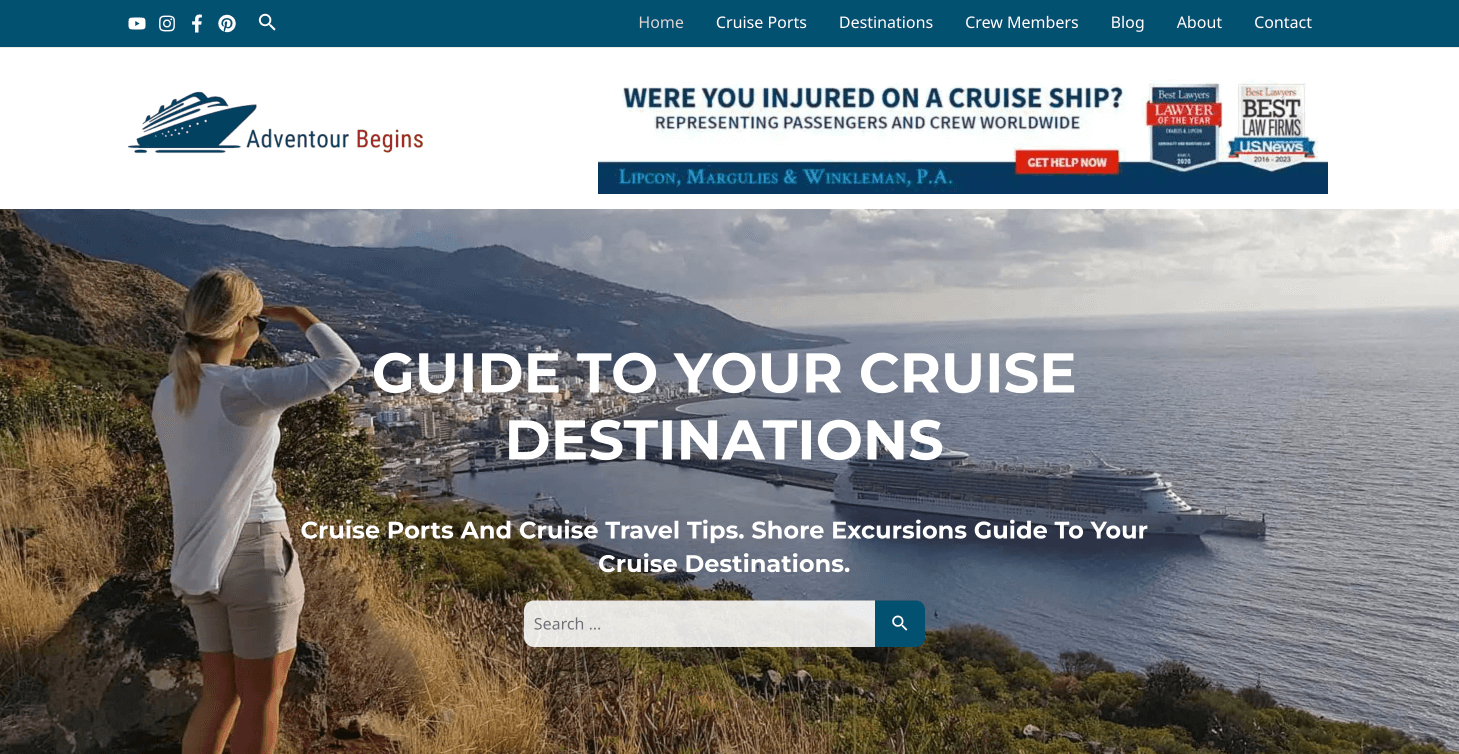This is a highly detailed screenshot of a web page titled "Adventure Begins," identifiable by its cruise ship icon in dark green, situated to the left of the page title. Adjacent to the title, on the right side, is a banner advertisement from the law firm Lipcon, Margulis, and Winklevin PA, which reads, "Were you injured on a cruise ship? Representing passengers and crew worldwide." The banner also features a prominent red "Get Help Now" button.

Below the banner, there is an image of a bay, capturing a woman standing on a hillside and looking out over the ocean. She is wearing a white shirt and beige shorts. The photo showcases a cruise liner traveling towards the right, with a small seaside town featuring numerous buildings near the coastline and nestled against the hillside. The sky is partly cloudy with a haze lingering on the horizon.

Overlaying this picturesque scene is white text that reads: "Guide to Your Cruise Destinations, Cruise Ports and Cruise Travel Tips, Shore Excursions Guide to Your Cruise Destination." At the bottom of the image, there's a small search bubble providing a tool for further exploration.